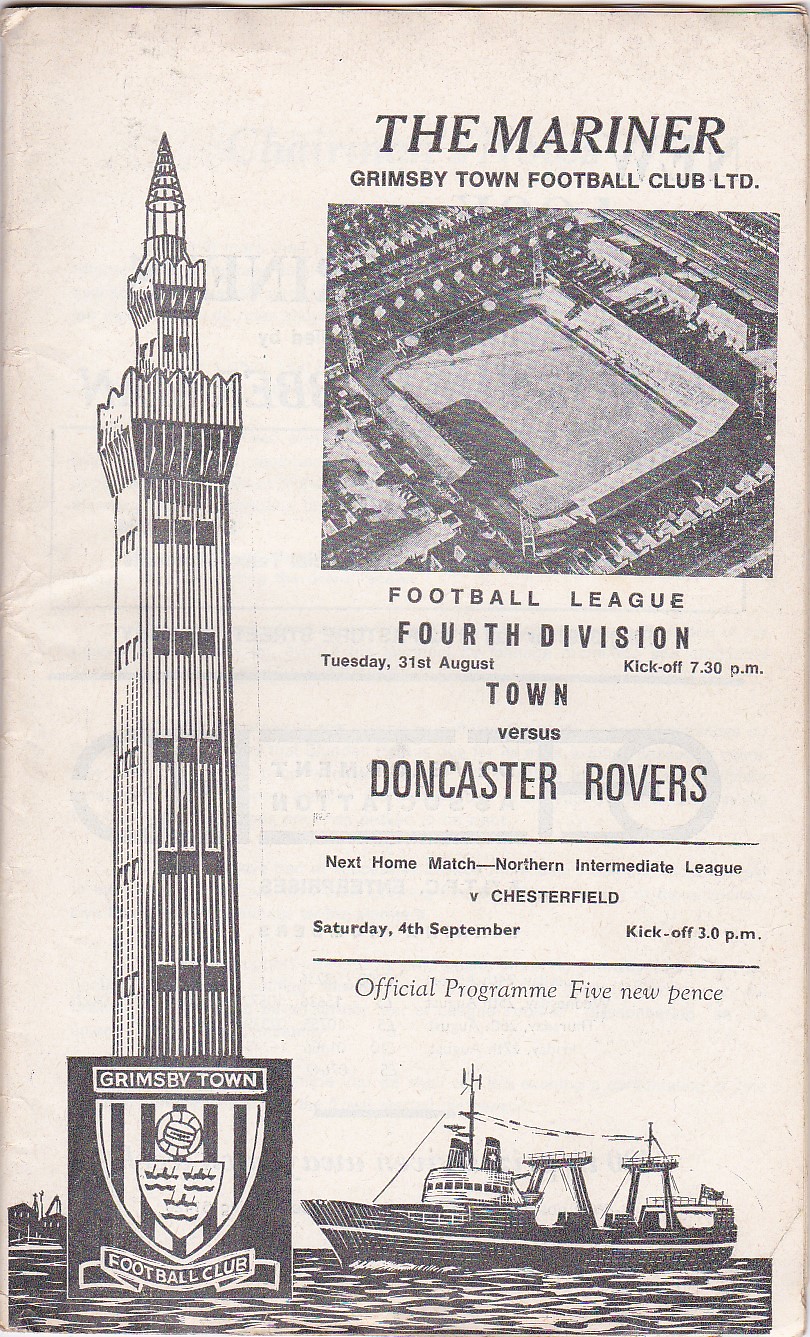We're looking at a detailed black-and-white brochure for the Mariners, associated with the Grimsby Town Football Club Limited. At the top, the heading reads "The Mariner," and below it is a picture of the stadium taken from a distance. The brochure announces the Football League, 4th Division match on Tuesday, 31st of August, with kickoff at 7:30 PM, featuring Grimsby Town vs. Doncaster Rovers. Below this, another highlighted section reveals the next home match in the Northern Intermediate League against Chesterfield, scheduled for Saturday, 4th of September, with a 3 PM kickoff. 

The official program section is titled "Five New Pens," a playful note hinting at new elements compared to the old. Adjacent to these announcements, there's an illustration of a cargo freighter with cranes at midships and stern, a wheelhouse with a prominent antenna, and a line of pennants stretching from the bow to the rear mast. Further to the left, an image shows a lighthouse-like obelisk with a railed platform near the top and a spire of metalworks extending into the sky. The entire brochure is designed in striking black ink on white paper, encapsulating the essence of the Grimsby Town Football Club.